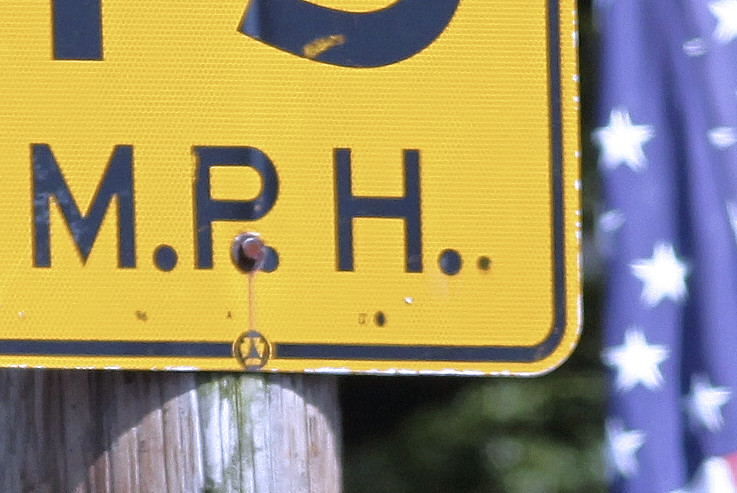This image captures the lower section of a street sign, presumed to be a speed limit sign, as evidenced by the partially visible letters "MPH" at the bottom. The sign is square, painted in a bright yellow hue with bold black lettering, and appears to be mounted on a vertical pole. The background is artfully blurred, highlighting the sign but allowing for a glimpse of an American flag. The flag's blue field adorned with white stars is clearly discernible, along with a hint of a red stripe peeking out from the lower corner of the frame, adding a patriotic touch to the scene.